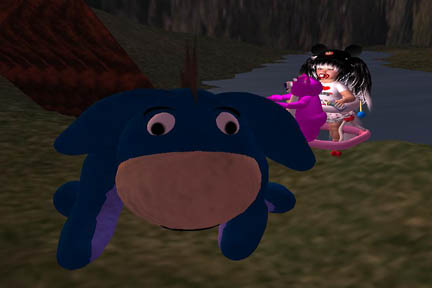In the image, we see a vibrant scene featuring animated video game characters. In the foreground, there is a character resembling a blue stuffed animal with distinct features: it has a pair of arms, a light brown, prominent nose, white eyes with black pupils, and expressive eyebrows. 

Standing slightly behind, there is a doll holding a purple teddy bear. The doll is dressed in a white shirt and has long black hair flowing down its back. The background showcases a natural setting with a brown tree stump situated to the left, a blue creek flowing to the right, and lush green grass covering the ground. The colorful and detailed environment brings the characters to life, creating an engaging and whimsical scene.